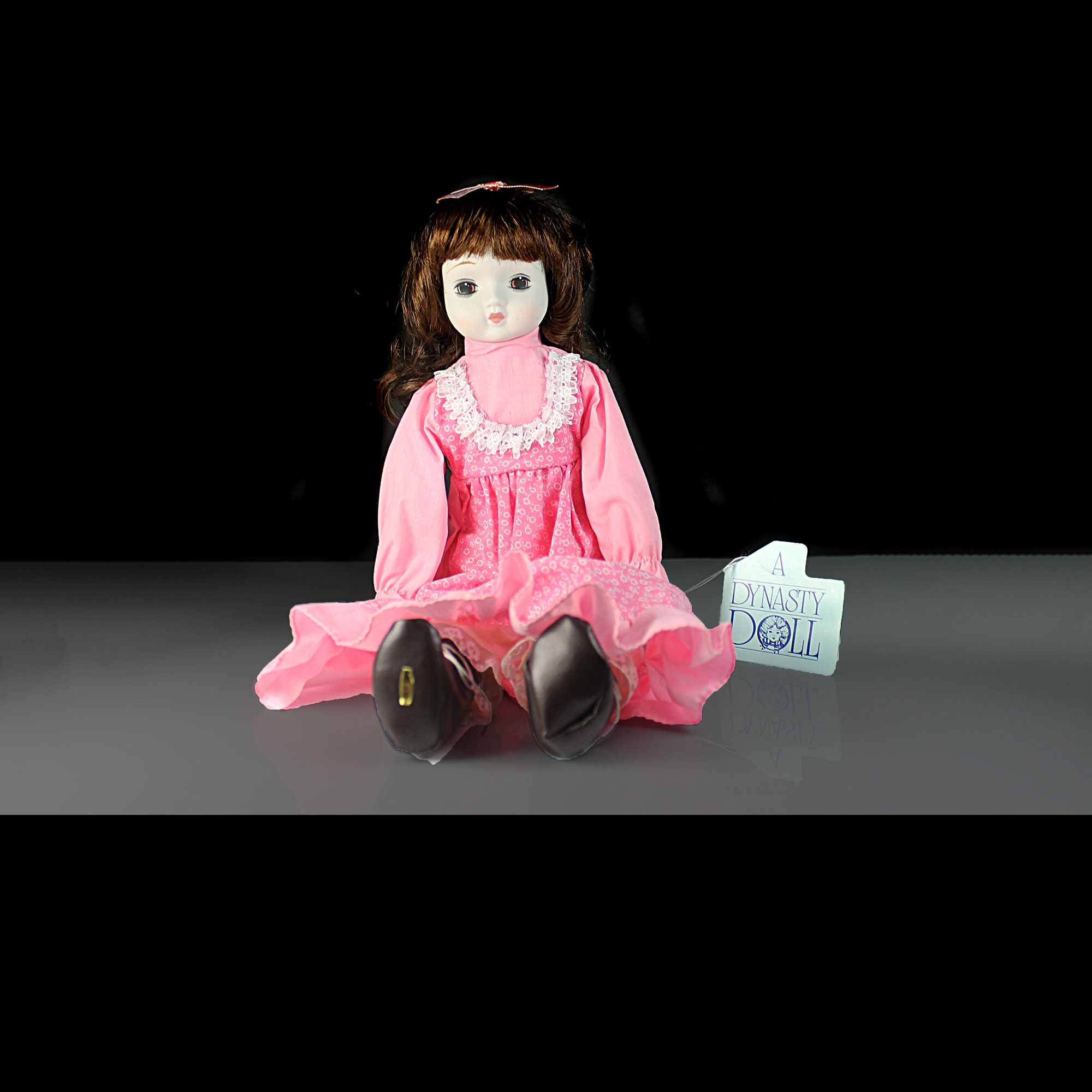The image features an antique ceramic doll with a white, pale face and distinct facial features, including light pink puckered lips. The doll has long, curly brown hair with straight bangs and a pink bow on top of its head. It is dressed in a long, pink, long-sleeved gown that reaches the floor and is adorned with white ruffles and lace detailing around the neckline and mid-chest area. The doll is seated on a gray shelf against a pitch-black background. Her black shoes, one with a golden sticker, are pointed towards the viewer. Next to the doll, there is a tag attached to its arm that reads "Dynasty Doll" in gold lettering.